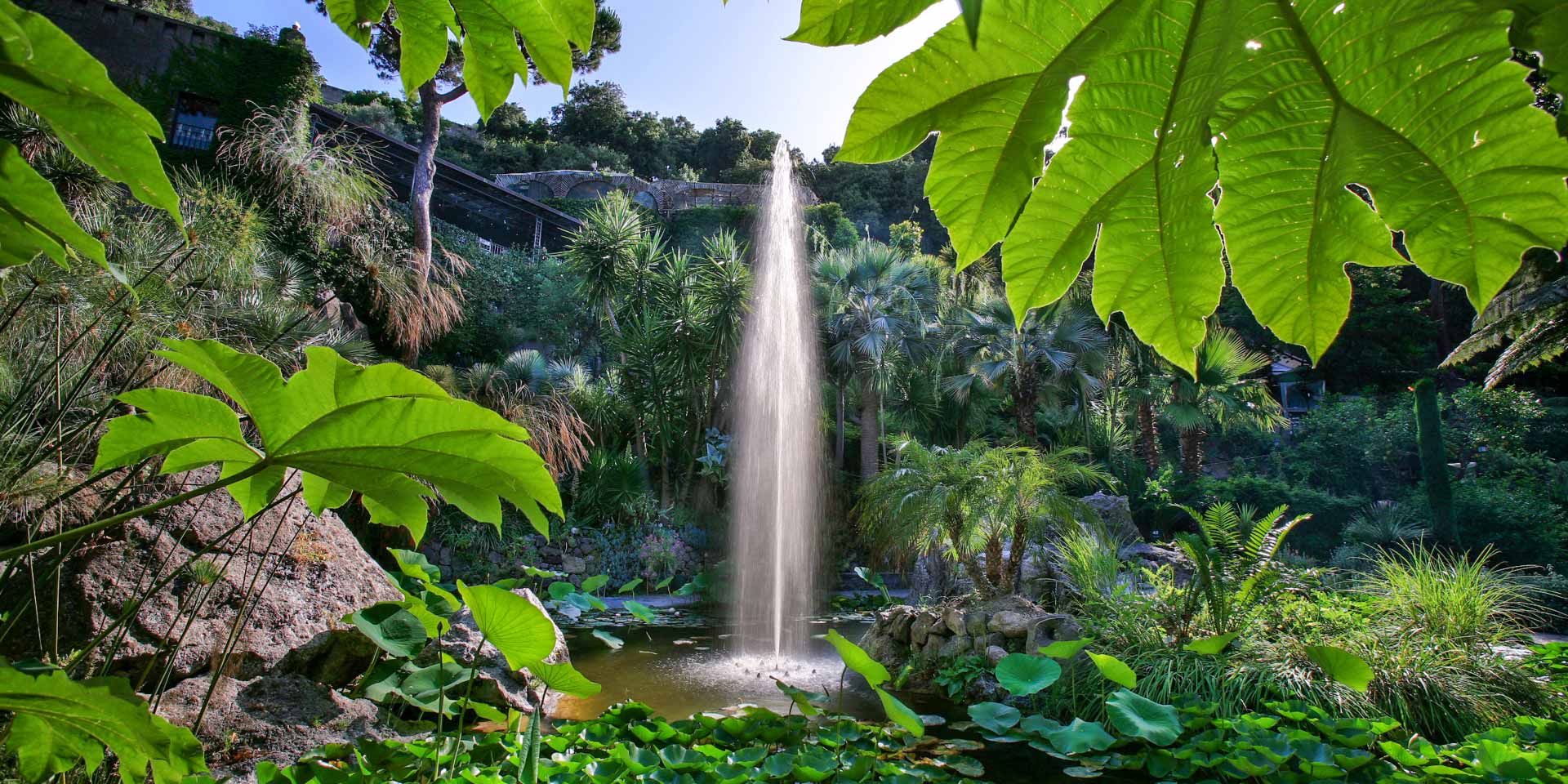The image is a detailed landscape photograph capturing a lush, tropical environment dominated by vibrant greenery. Prominently in the center, a thin fountain or geyser shoots a high, misty stream of water at least 20 feet into the air, tapering to a point before broadening as it cascades back down into a small, greenish pond. This pond occupies the lower quarter of the image, surrounded by tall, bushy ferns, leafy plants, and water plants, adding to the jungle ambiance.

On the upper right corner, an expansive green leaf intrudes into the frame, mirrored by similar foliage in the lower left. The backdrop rises into a rocky, hilly terrain dotted with large boulders and slopes upward, revealing a mix of tropical plants, including palm trees and towering green shrubs. To the left side, there’s a rocky embankment with clusters of broad leaves and a large boulder. Trees and additional tropical flora hint at the borders of a cliff or hill.

In the very background, you find a light blue, clear sky with no clouds, adding contrast to the dense greenery. There's also an impression of man-made elements, including a concrete structure, possibly a bridge with a ladder leading up and details of what appears to be a tent atop the hill. This adds a sense of depth and human presence to the otherwise natural scene.